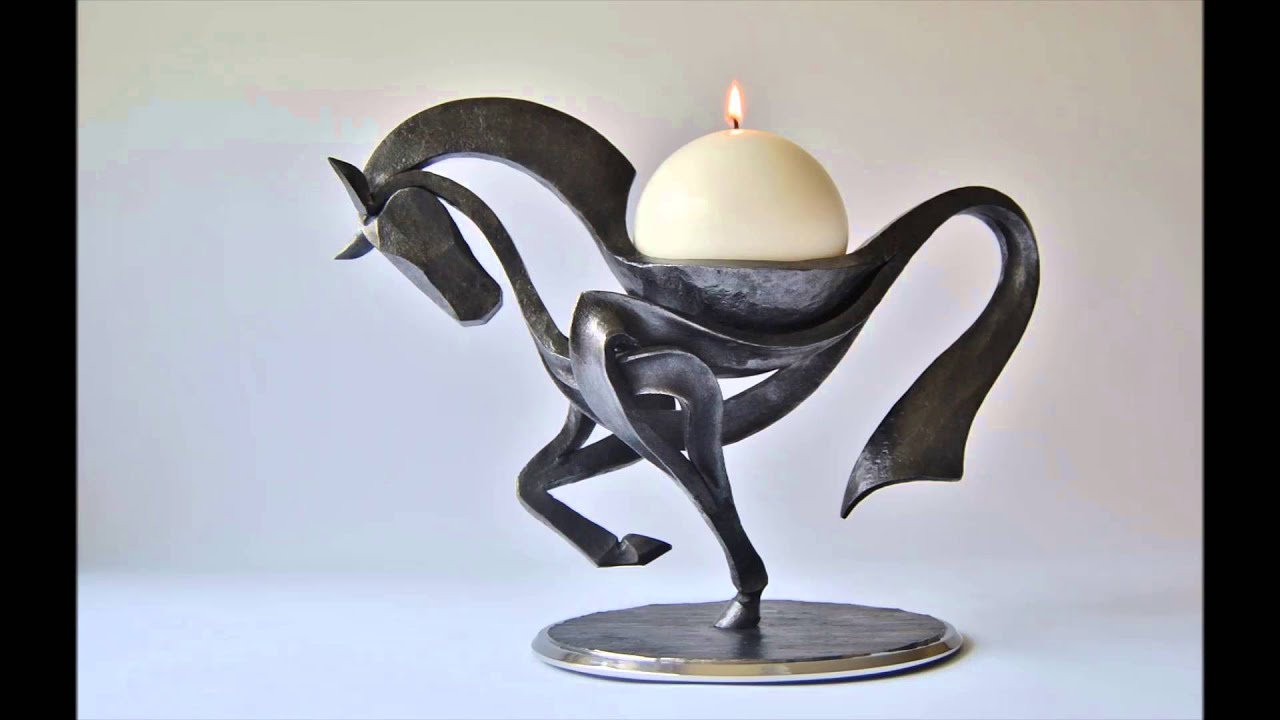This photograph showcases an intricately designed, modern artistic candle holder in the form of a two-legged horse, predominantly black in color with a smooth, metallic finish, possibly made of bronze or a stone-like material. The horse is depicted standing on a pale blue circular base, supported by one of its forelegs while the other is lifted in a striking pose. It has a gracefully curved neck with its head bent downward and a thick, s-shaped tail extending elegantly behind it. Centered on the horse's back is a round, white, scented candle, which is lit and emanates a warm orange glow. The image is set against a bluish-purple background with black borders on the sides, suggesting an indoor setting that's part of sophisticated interior decoration.